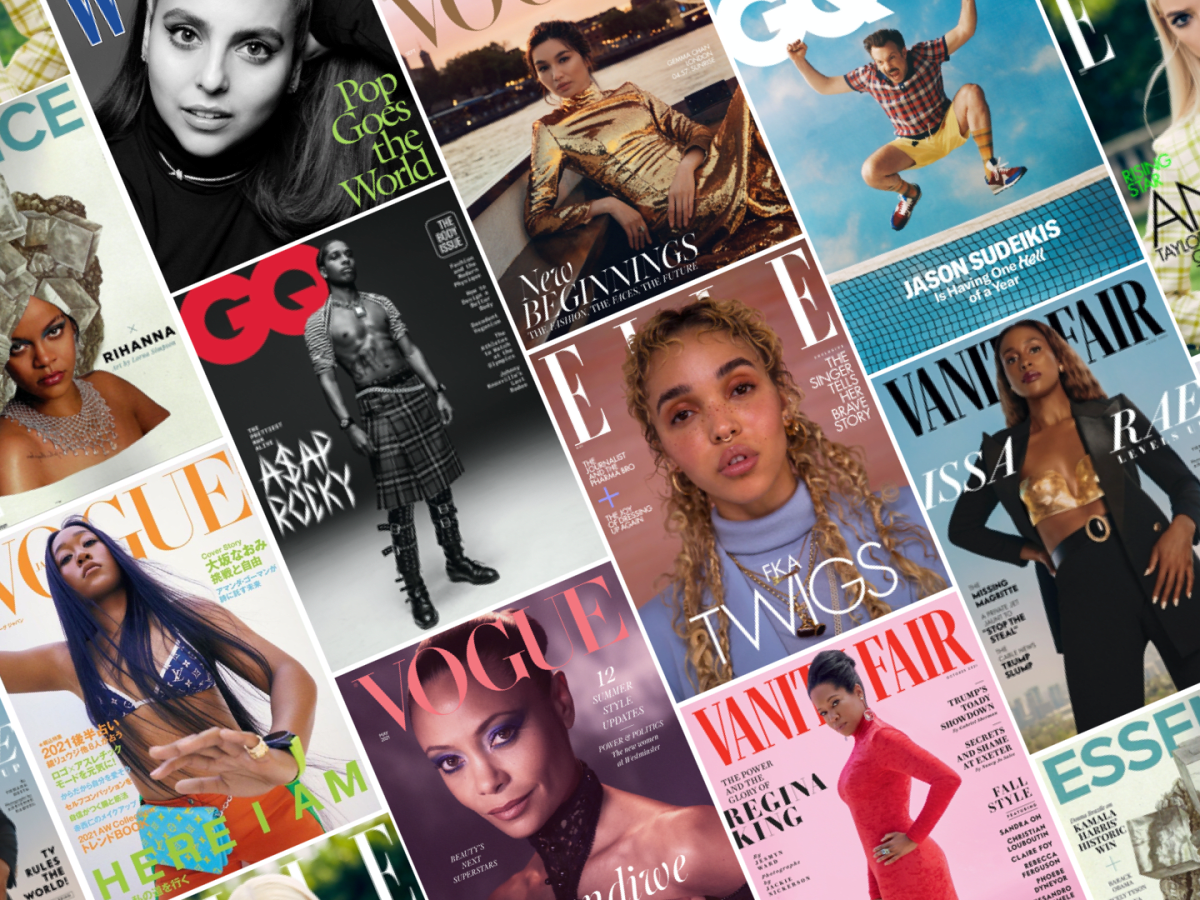The image features a diagonally aligned collage of various contemporary fashion and lifestyle magazine covers, spread across the ground and canted slightly to the left for an interesting visual effect. Among the noticeable magazines are multiple issues of Vogue, Essence, and Vanity Fair. The covers showcase a diverse array of figures: Rihanna adorned in a Ming Jewel necklace on Essence, Jason Sudeikis on GQ, and ASAP Rocky on another GQ issue. Additional covers include FKA Twigs with distinct makeup and jewelry on Elle, and Gina King in a red dress on Vanity Fair. The collage also includes an Elle magazine with a mysterious partial cover, possibly of another high-profile individual. The vibrant mix of colors and titles creates a scene reminiscent of a newsstand display, capturing a slice of contemporary pop culture.